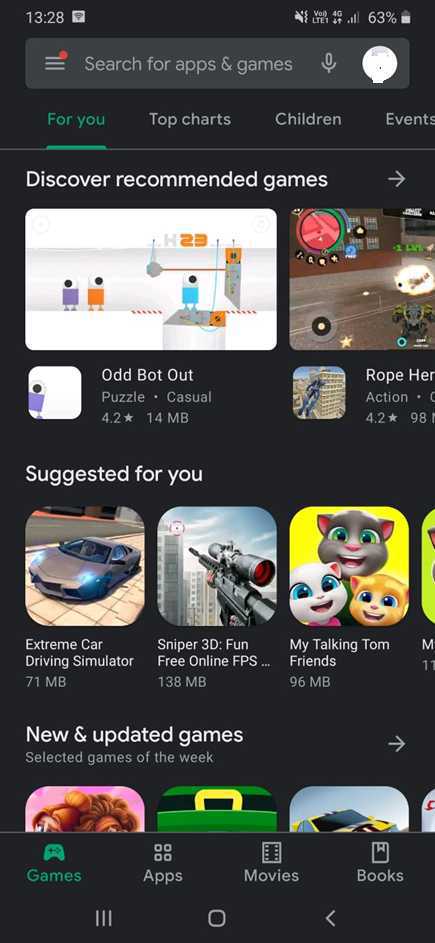A vertical screenshot taken from a smartphone displays an app store interface against a solid black background. The upper-left corner shows the time as 13:28, while the upper-right corner features white icons indicating Wi-Fi signal, network strength, sound status, and a battery life of 63%. Below this, a gray search bar is visible for finding apps and games. 

The highlighted tab in green reads "For You," accompanied by other tabs labeled "Top Charts," "Children," and "Events." A line separates these tabs from the content below, which begins with "Discover Recommended Games." This section features various game icons, titles, categories, star ratings, and space requirements. Following this, under the "Suggested for You" category, it continues with a similar layout of game details.

Further down, the "New and Updated Games" section highlights selected games of the week, though some images are partially cut off. At the bottom of the screen, the "Games" tab is highlighted, alongside icons for "Apps," "Movies," and "Books." Additional app-related icons are seen at the very bottom of the image.